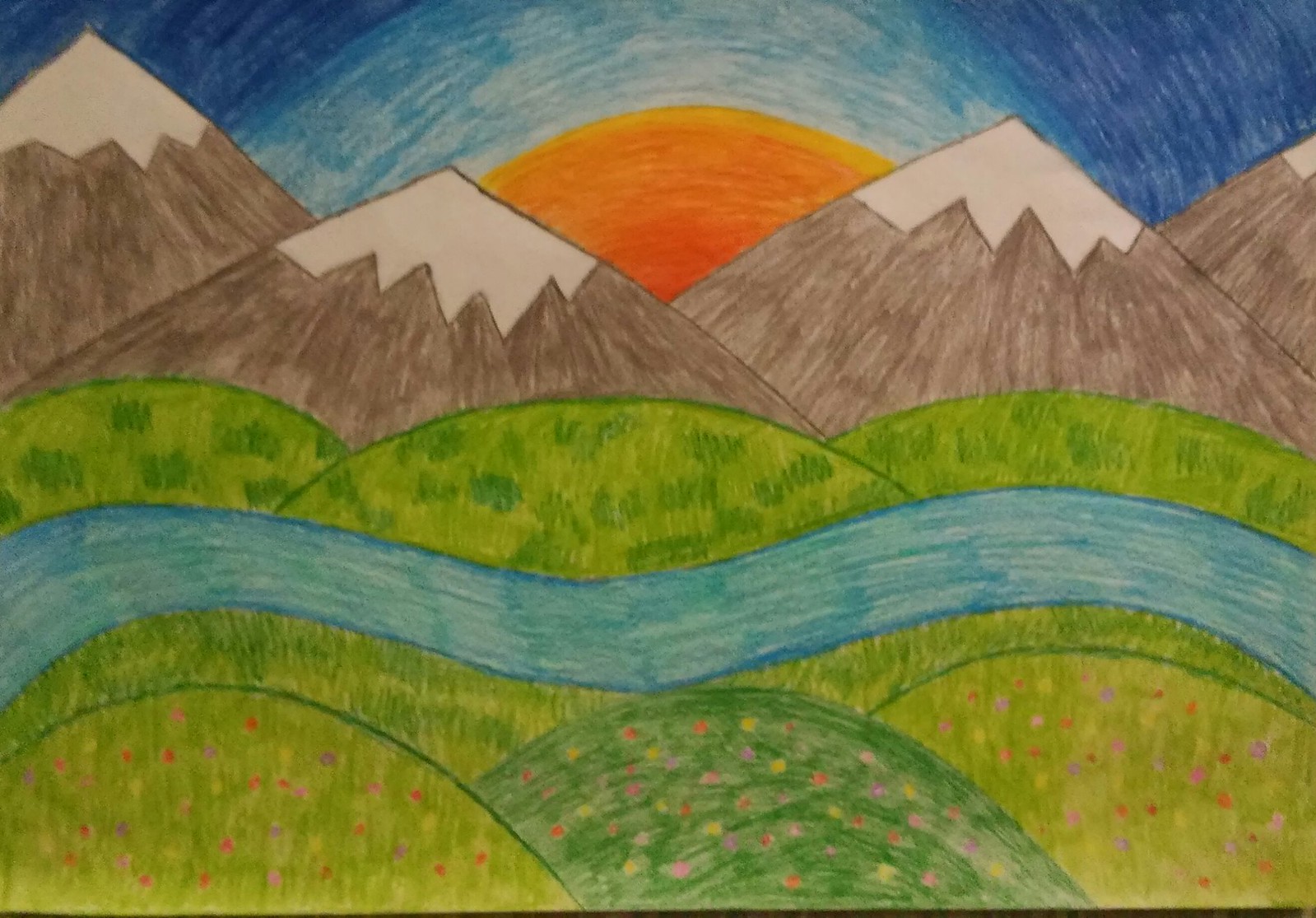This artwork is a vibrant drawing of a serene meadow with a winding stream, set against a backdrop of majestic mountains and a radiant sun either rising or setting. The drawing employs a series of overlapping semicircles to artistically represent rolling hills and mountainous landscapes. The stream is depicted in a vivid blue, while the mountains are a rich brown capped with snowy white peaks. The sun is harmoniously colored with shades of gold, yellow, and orange, adding warmth to the scene. The sky features two distinct shades of blue, with a lighter hue indicating daylight and a darker blue signifying night. The entire piece, seemingly created with markers, showcases a dynamic range of colors and textures, highlighting the artist's keen eye for detail and creativity.